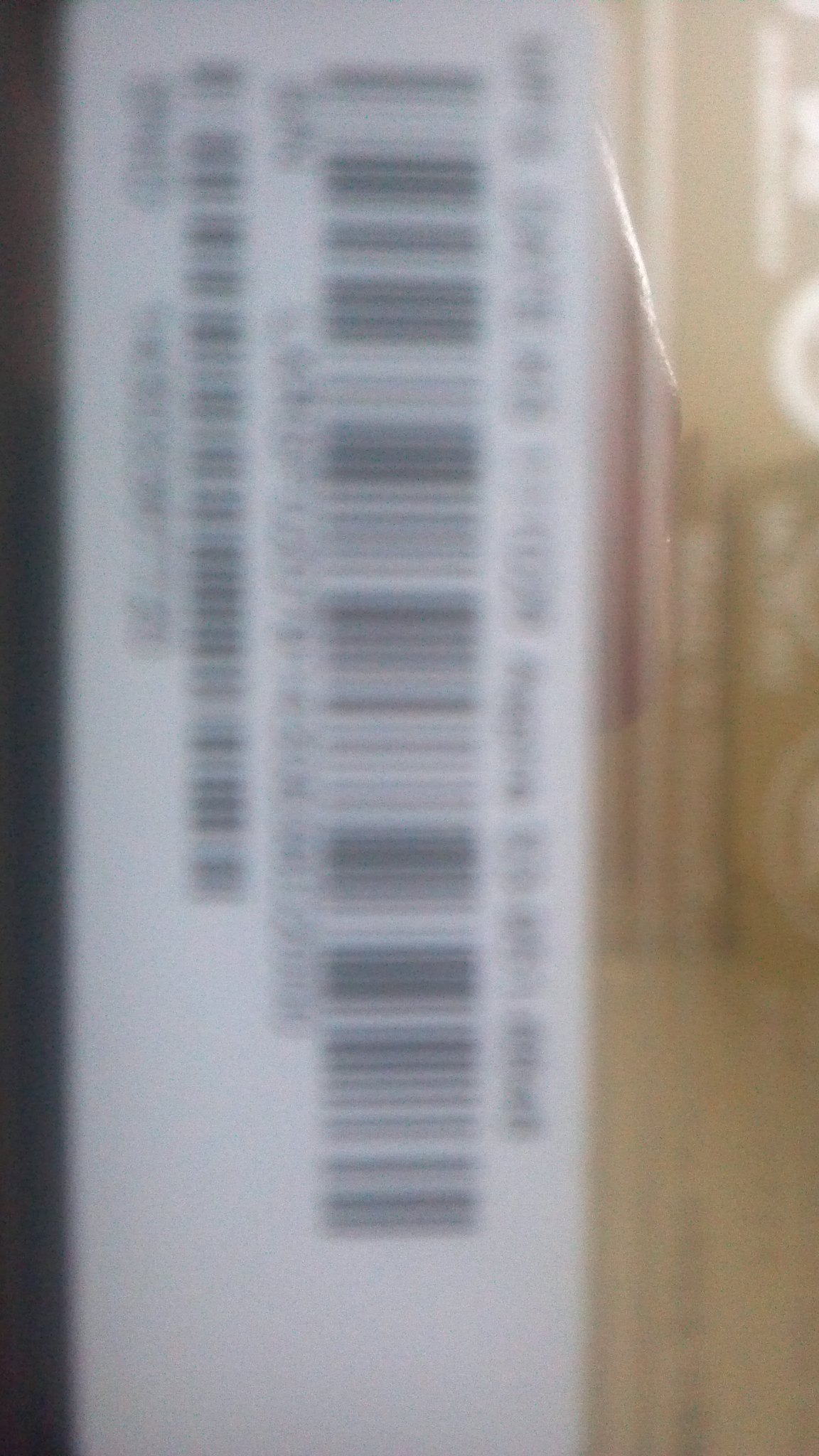The image is a color photograph featuring an extreme close-up of a label on a package, which is completely out of focus and blurred. The label, likely affixed to a brown cardboard box, predominantly showcases a series of barcodes on a white background. Although the content is obscured due to the blur, a few visual cues remain discernible: the label contains two primary barcodes, described as a wider and deeper barcode across the middle, accompanied by a few numbers followed by a series of barcode numbers, and a narrower, shorter barcode beneath it, likewise followed by a string of characters. Given the orientation of the label in the photograph, it appears to need a 90-degree anti-clockwise rotation to be correctly aligned. Sparse, illegible text and numbers are visible above and below these barcodes. Additionally, the edges of the photograph include hints of a light brown background, potentially the cardboard box, and a vague, shadowy figure towards the left.